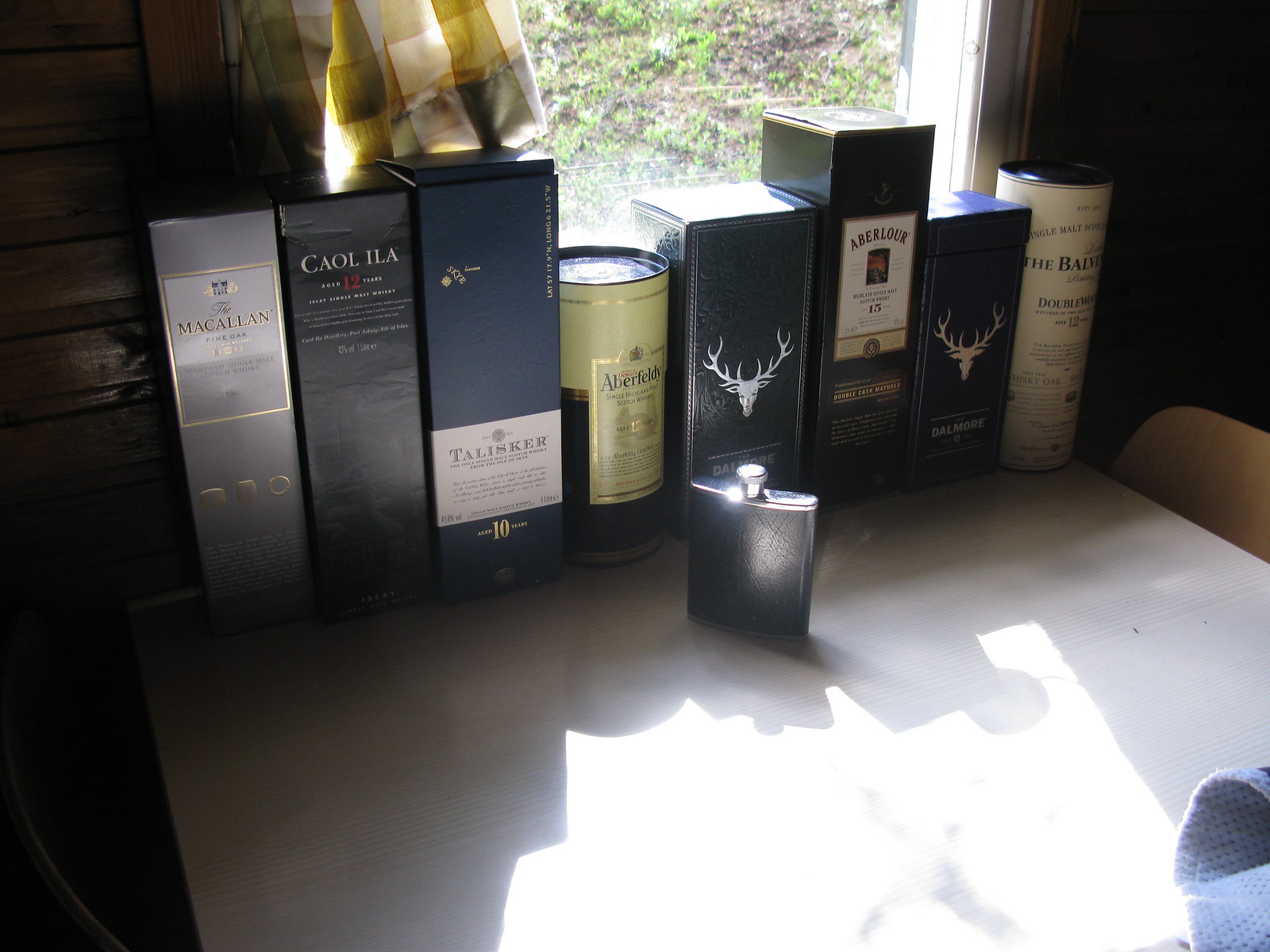The image depicts a detailed scene centered around a white table. In the bottom right corner of the table, a waffle-patterned piece of cloth is visible. Two brown wooden chairs are pushed in under the table on either side. The table is laden with a collection of alcohol boxes, varying in shapes—some rectangular, others cylindrical—and brands including Macallan, Talisker, Aberfeldy, Cowell-Ela, Dalmore, Abelour, and partially visible, The Balvenie. A square-shaped flat metal flask with a silver cap sits prominently on the table in front of the boxes. At the end of the table, a window covered with an open yellow and white plaid curtain reveals a yard with green vegetation and brown patches of dirt.